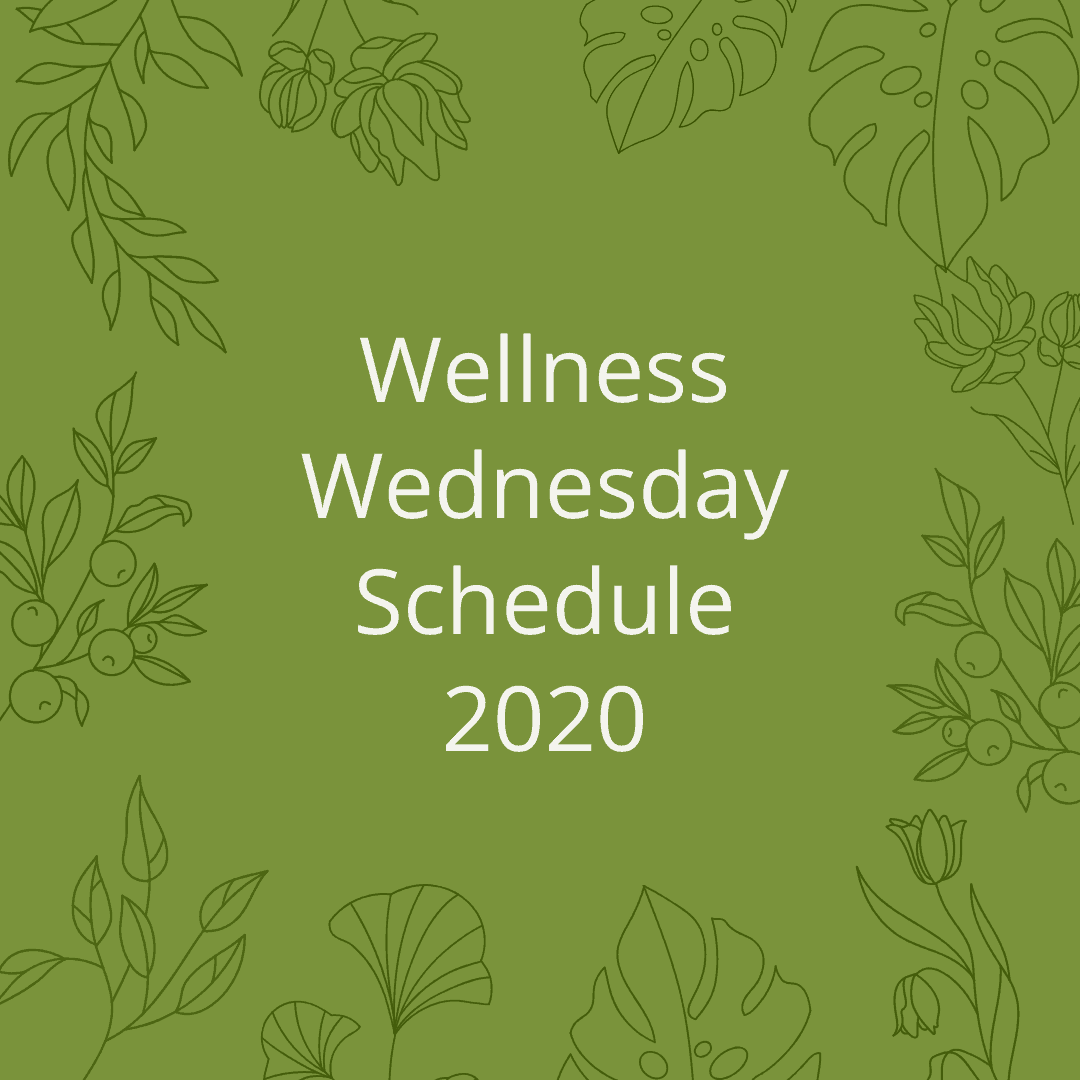The image presents an unclear setting, as it could be displayed on a website, mobile tablet, desktop, or browser. Dominated by an olive green square background, the image prominently features the text "Wellness Wednesday Schedule 2020" in large, white title-case letters. However, no schedule details are visible within the image. Stylized black outline illustrations of various plants and flowers, such as thistles, monstera leaves, carnations, tulips, olives, and berries, adorn the periphery of the green square. These illustrations frame the text, though their lack of color makes plant identification challenging. The overall design creates a decorative border around the central text.